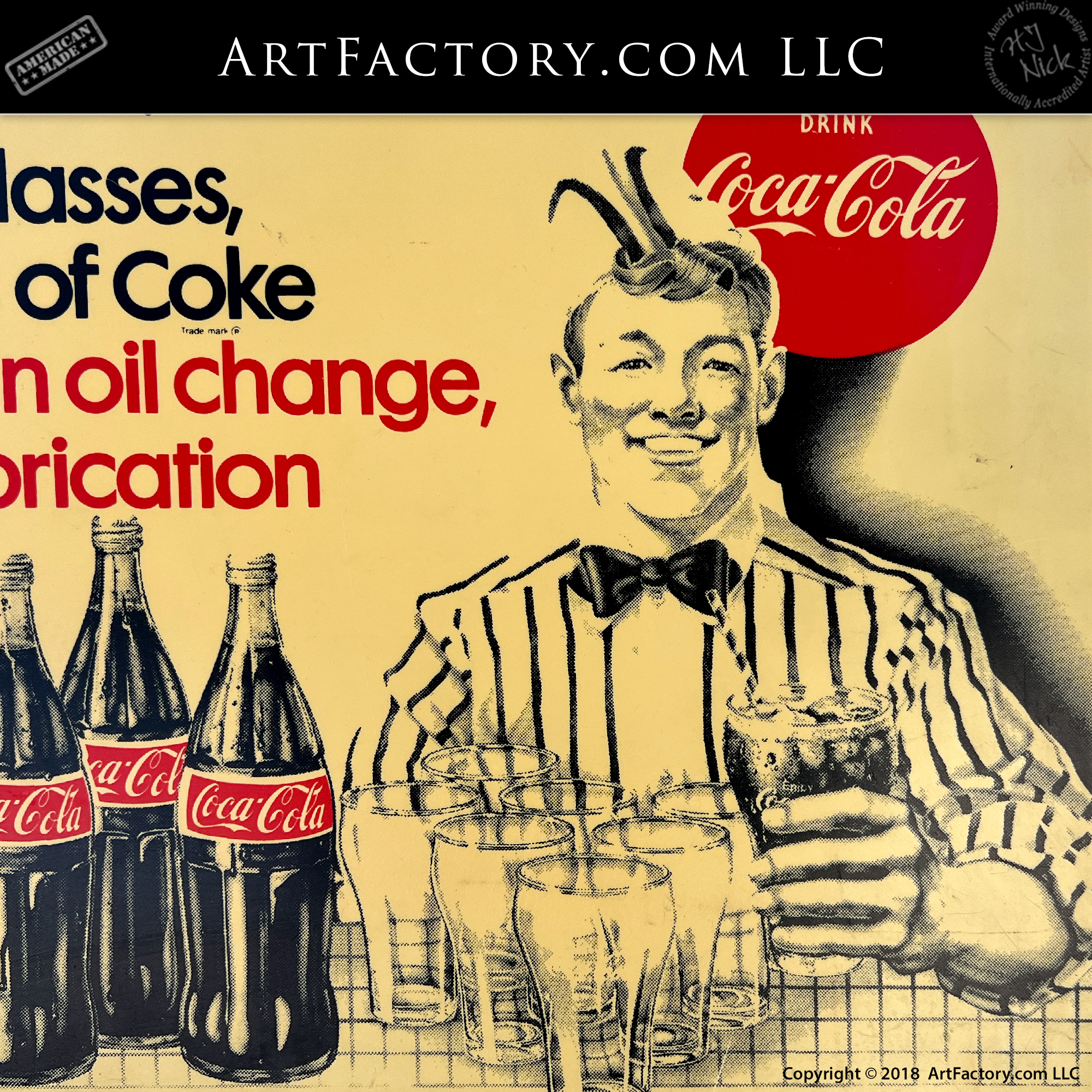The image is a promotional advertisement with a predominantly dark yellow background. It has a square format with a distinct black banner at the top that reads "ArtFactory.com LLC" and "American made." Below the banner, on the right side, there's a prominent red circle featuring the "Drink Coca-Cola" logo. The ad centers on a cheerful man attired in a classic soda jerk uniform, complete with a striped jacket, bow tie, and a classic soda jerk hat. His image is depicted in yellow and black tones, accentuating the vintage feel. He smiles toward the camera, holding up a glass filled with ice, Coca-Cola, and a straw. In front of him on the table, there are seven empty glasses, and to the bottom left, three traditional glass bottles of Coca-Cola are noticeable. To the left of the man, text in black reads "Glasses of Coke," and in red, it says "Oil Change Lubrication." At the bottom of the ad, it mentions "Copyright 2018 ArtFactory.com LLC."